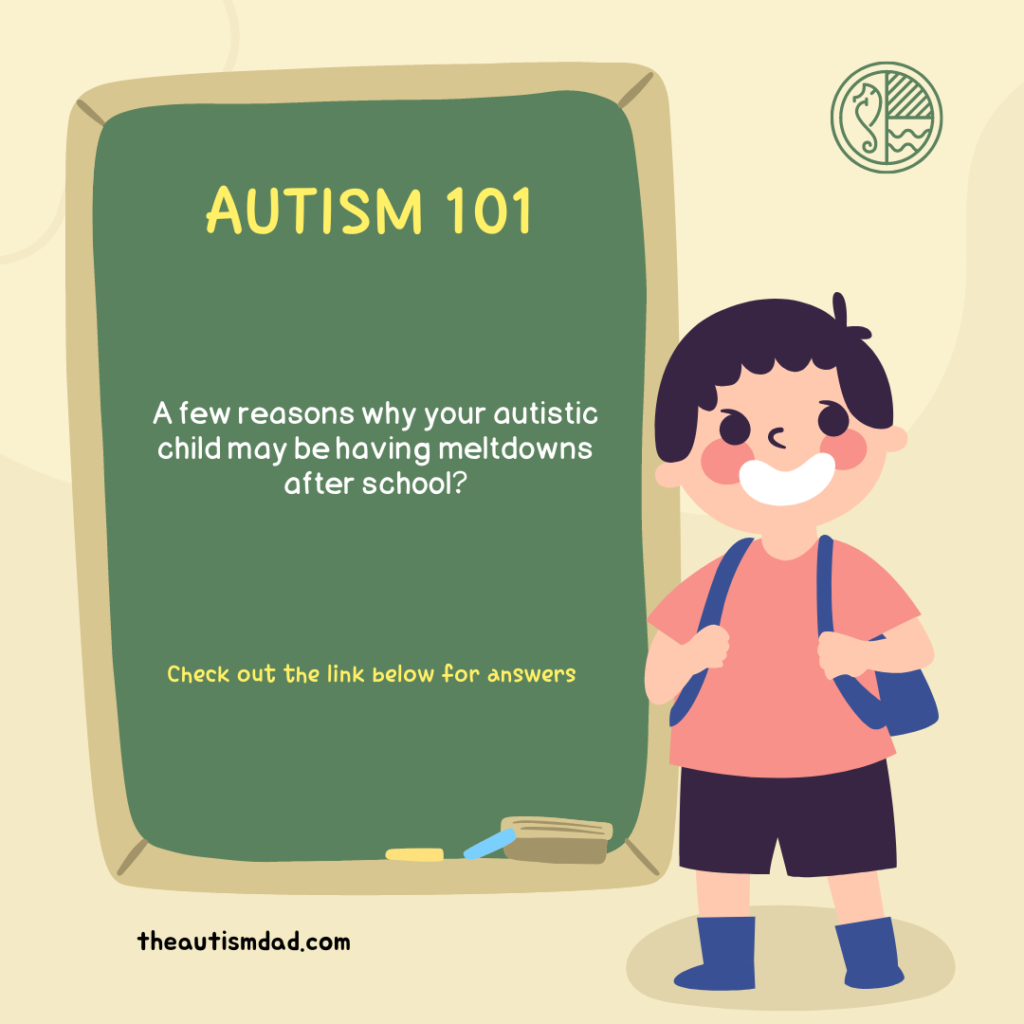The illustration is an educational piece providing information about autism. In the image, on the right side, there is a cartoon drawing of a smiling boy with short black hair. He wears a salmon-colored shirt, black shorts, blue boots, and a blue backpack, which he is holding onto with each hand. To his left, there is a vertically oriented green chalkboard with a cream-colored frame, designed to look like a classic school chalkboard. The chalkboard displays the title "Autism 101" in large yellow letters at the top. Below that, in smaller white text, it reads, "A Few Reasons Why Your Autistic Child May Be Having Meltdowns After School?" At the bottom of the chalkboard, in smaller yellow letters, it instructs viewers to "Check Out the Link Below for Answers." Underneath the chalkboard, in black lowercase letters, is the URL "theautismdad.com." The background of the illustration is yellowish, and a small circular logo featuring a seahorse is located in the upper right corner of the image. The illustration aims to direct viewers to the website for more information.